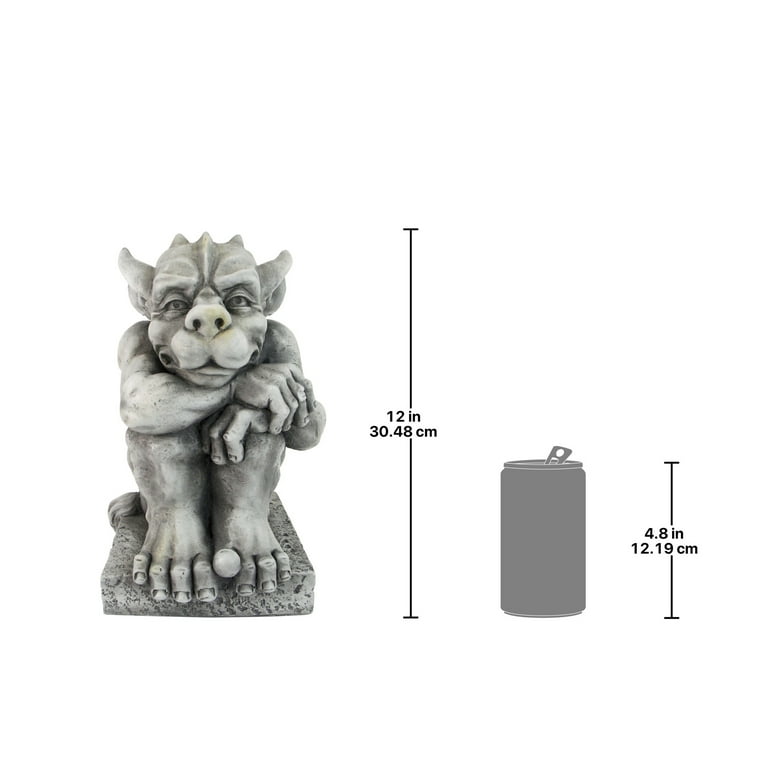The image depicts two objects with a scale of measurement beside each. On the left side, there is a detailed statue resembling a gargoyle. The creature, light green and gray in color, has a unique appearance with somewhat pointed ears, small horns atop its head, and large, prominent nose and mouth. It is crouched with its right arm resting across its body on its left wrist, which in turn is braced on its left knee. Notably, the big toe on its right foot is raised above the other toes. The creature is positioned on a simple square flat pedestal and seems to be looking directly forward. Above its head, a tail is slightly visible extending to the left side. To the right of the statue, a vertical black line with small horizontal lines at both ends shows its height – 12 inches or 30.48 centimeters.

To the far right, there is an image of a gray soda can with its tab up. Adjacent to the can is another vertical black line with small horizontal lines at the top and bottom, indicating the can's height – 4.8 inches or 12.19 centimeters. The background of the entire image is solid white, creating a bright and clear setting that enhances the visibility and detail of both the gargoyle statue and the soda can. This comparison highlights that the gargoyle is much larger than the soda can.